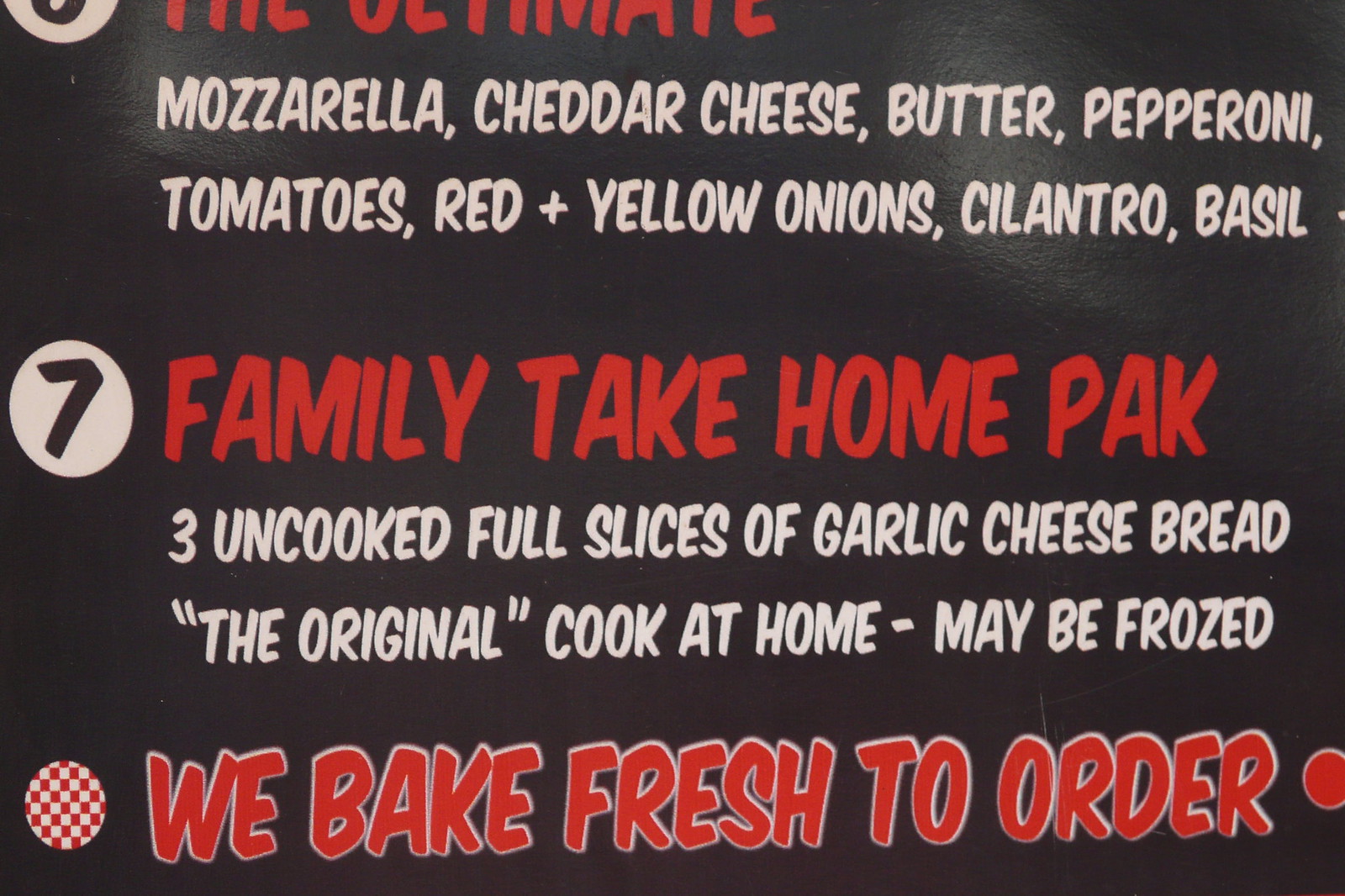The image depicts a close-up section of a black menu board with both red and white text. At the very top, partially cut off, the number six is visible alongside a red word that isn’t fully captured in the image. Below it, a list of ingredients is written in white text: mozzarella, cheddar cheese, butter, pepperoni, tomatoes, red and yellow onions, cilantro, and basil. Underneath, the menu continues with a white circle encasing a black number seven. Adjacent to this, in bold red letters, it reads "Family Take-Home PAK." Following this, white text details the offering: "Three uncooked full slices of garlic cheese bread." In quotes, it states "The original cook-at-home – may be frozed." Further down in large red letters with a white outline, the menu proclaims "WE BAKE FRESH TO ORDER." To the left, a red and white checkerboard circle adds a decorative element, and to the right, a small red dot punctuates the end of the text. The overall background of the image is black, emphasizing the bright red and white text.